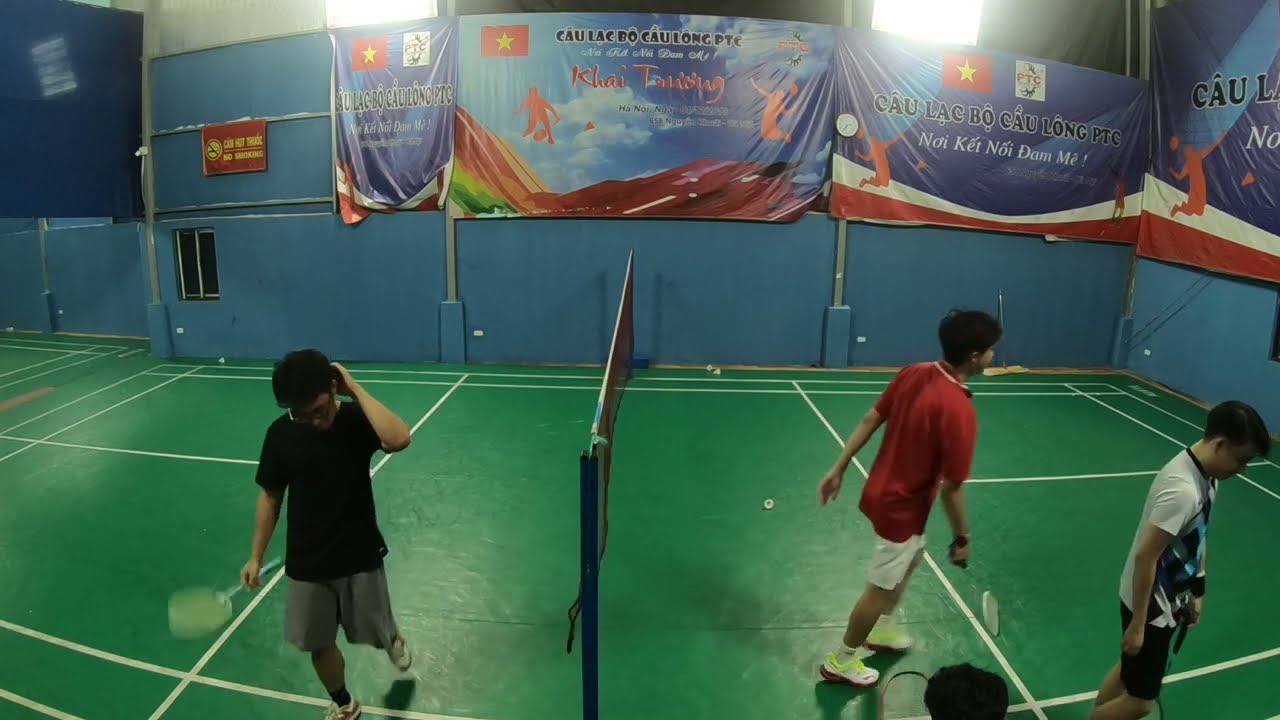This is a detailed photograph of an indoor tennis court taken from the side, capturing a dynamic scene of a doubles match in action. The green court is marked with white lines and separated by a central net. On the left side of the net is a young male player of Asian descent, wearing a black t-shirt and gray shorts. He has glasses and appears to be looking down, holding a tennis racket. On the right side of the net are two other young male players, also of Asian descent; one is dressed in a red shirt with white shorts, while the other wears a white shirt with blue accents paired with black shorts. Both players on the right are also holding tennis rackets. The players seem to be in their teens or early twenties. Encircling the court is a blue border or wall, above which colorful signs with reds, blues, and yellows are displayed, adorned with flags and stars. These signs are written in a foreign language, adding an international flair to the indoor setting.